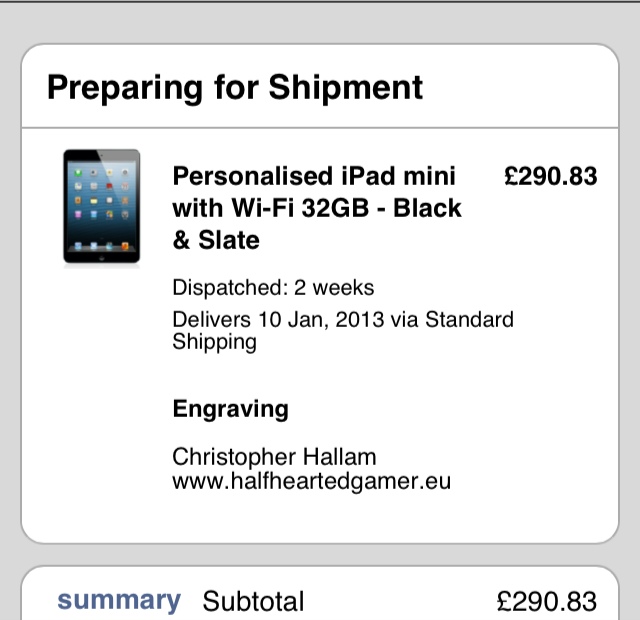The screenshot, likely taken from a mobile phone (possibly an iPhone), depicts a shipment notification for an Apple device. The background of the screenshot is light gray with a prominent white square featuring rounded corners occupying most of the image. At the top of this white square, large black text reads "Preparing for Shipment," with a gray horizontal rule beneath it. On the left side of the square, there's a color photo of an iPad. Next to the photo, the text details a "Personalized iPad mini with Wi-Fi, 32 gigabytes, Black and Slate" priced at £290.83. The shipment is marked as dispatched in two weeks, set to deliver on January 10, 2013, via standard shipping. The engraving reads "Christopher Hallam" along with the URL "www.halfheartedgamer.eu." Below this section, a summary indicates a subtotal of £290.83, though part of this white box is cropped off in the screenshot.